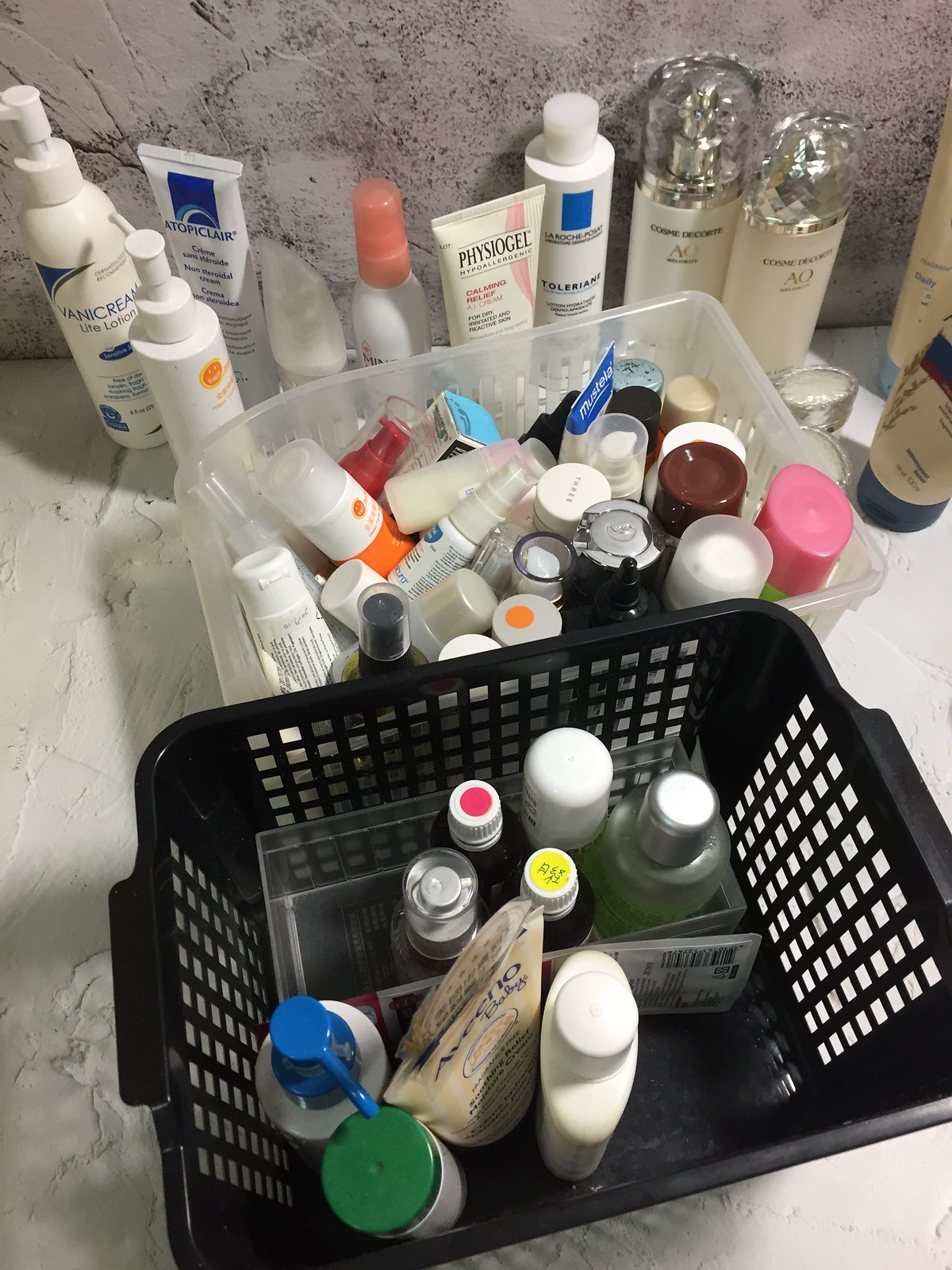The image showcases a heavily cluttered bathroom counter laden with an assortment of beauty and bath products. The countertop appears to be made of white marble, accented with darker gray marbling, although the abundance of items partially obscures the surface. The background wall, which also seems to be marble but in a slightly different shade, might be part of the shower area, though it is difficult to discern clearly.

Positioned against this marble backdrop are eleven bottles and tubes of creams, including identifiable brands such as Vanicream and Physiogel, suggesting a focus on skincare products. Directly in front of these bottles is a clear basket holding numerous smaller-sized products, some of which appear to be trial sizes. This basket contains an estimated total of 22 items, mostly organized vertically with their tops visible, featuring predominantly clear or white caps—though a few are highlighted with pink and maroon tops.

In front of this clear basket is a black basket holding fewer items, precisely nine in total. These items are predominantly bath products, with one easily recognizable brand being Aveeno. The photograph mainly captures the tops of the bottles, adding to the impression of a well-stocked but disorganized collection of personal care items.